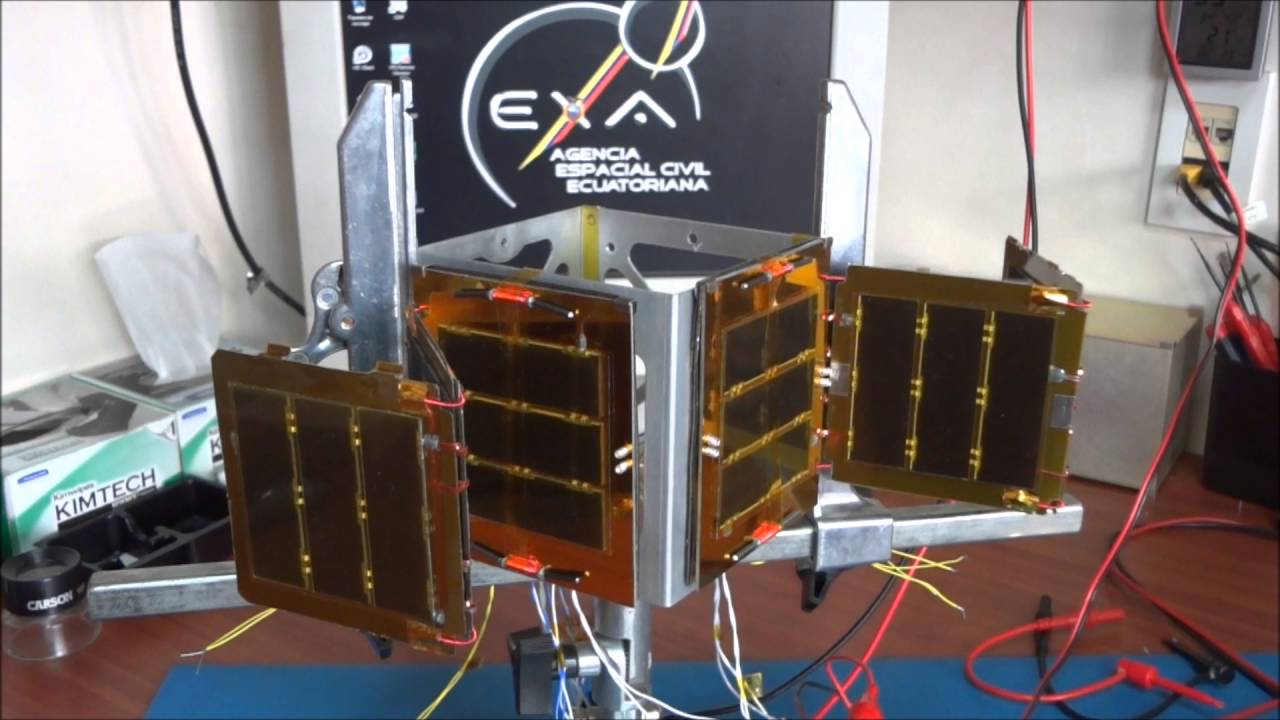The image depicts a cluttered room with a dark red wooden floor, featuring a scientific contraption prominently placed on a blue mat. The device is a metallic cube with open top and bottom, adorned with gold, solar panel-like plates on each side, and equipped with additional gold plates that extend outward, resembling wings. This machine, connected by a myriad of red and black wires, is plugged into two of the four outlets visible on the wall. Behind it, there is a black poster with the logo and text "EXA AGENCIA ESPECIAL CIVIL ECUATORIANA," denoting its Ecuadorian space agency origin. On the left, there are two boxes labeled "Kim Tech," one seemingly depleted, and possibly containing large tissue-like papers, with a black container in front of them. The room also contains a digital display that might be showing temperatures in Celsius, adding to the experimental atmosphere. The overall image quality is low, making some details blurry.